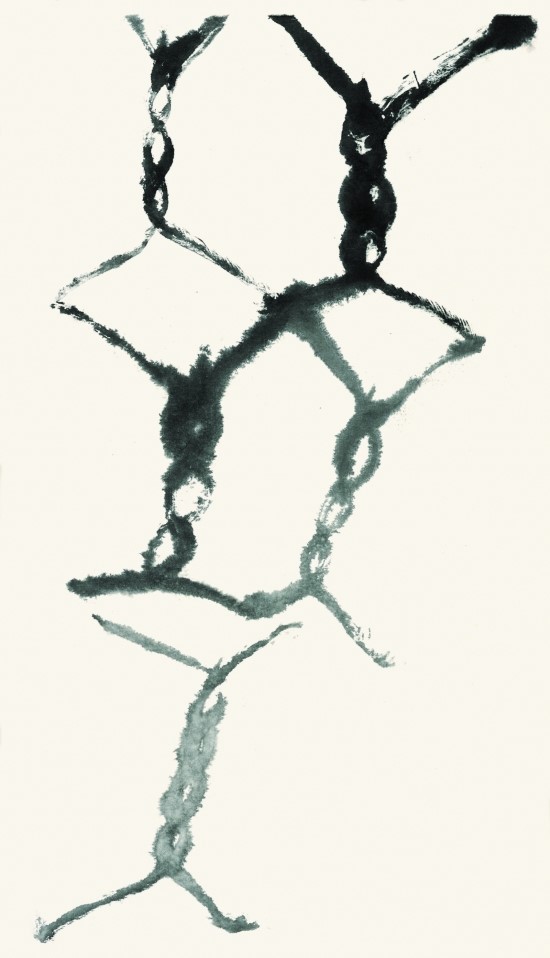The image appears to be an abstract artwork in a vertical rectangular format with an off-white to light pink background that provides a soft contrast. The primary elements within the image are repeated, twisted strands that resemble chains or wire, depicted using what seems to be black ink due to the blurred and feathery outlines of the lines. These strands or links show various figures or shapes – some forming diamond patterns or martini-glass-like forms. The strands are predominantly black and gray, with darker ones concentrated near the top and middle left sections, while lighter shades appear towards the right and bottom. These twisted figures create a mesh-like appearance similar to a chain-link fence, though they also evoke images of outstretched figures, possibly in gymnastic poses. The overall effect is a composition of intertwined, fuzzy, and detailed wires or chains against a minimalistic background, providing a complex yet cohesive visual structure.